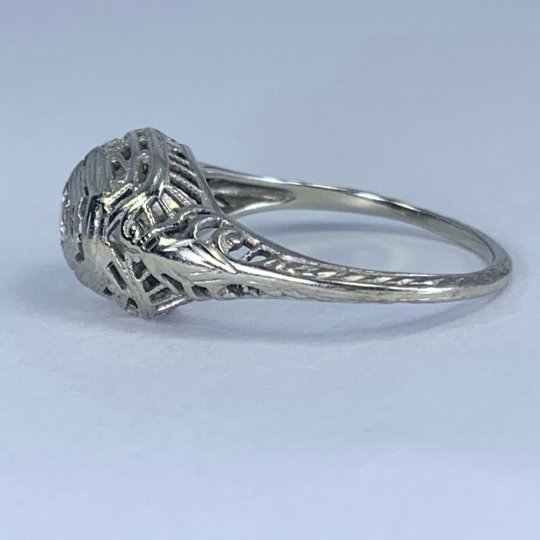This is an image of a silver ring, centrally positioned on a flat surface. The background transitions from a darker blue at the top to a lighter blue towards the bottom. The gem or embellishment part of the ring is facing to the left while the band is directed to the right. The ring itself is a sterling silver hue, thin in band, adorned with intricate etchings and slits that resemble small windows, giving it a breathable appearance. The main feature of the ring is a detailed silver mound, possibly a football helmet, suggesting it might be a sports-related ring, though not likely a Super Bowl ring. The design includes vertical engraved shapes and cutouts, adding to the ring's complex and precise craftsmanship. The ring lays flat on the table, with its engravings and rectangular cutouts contributing to a sophisticated yet sporty aesthetic.